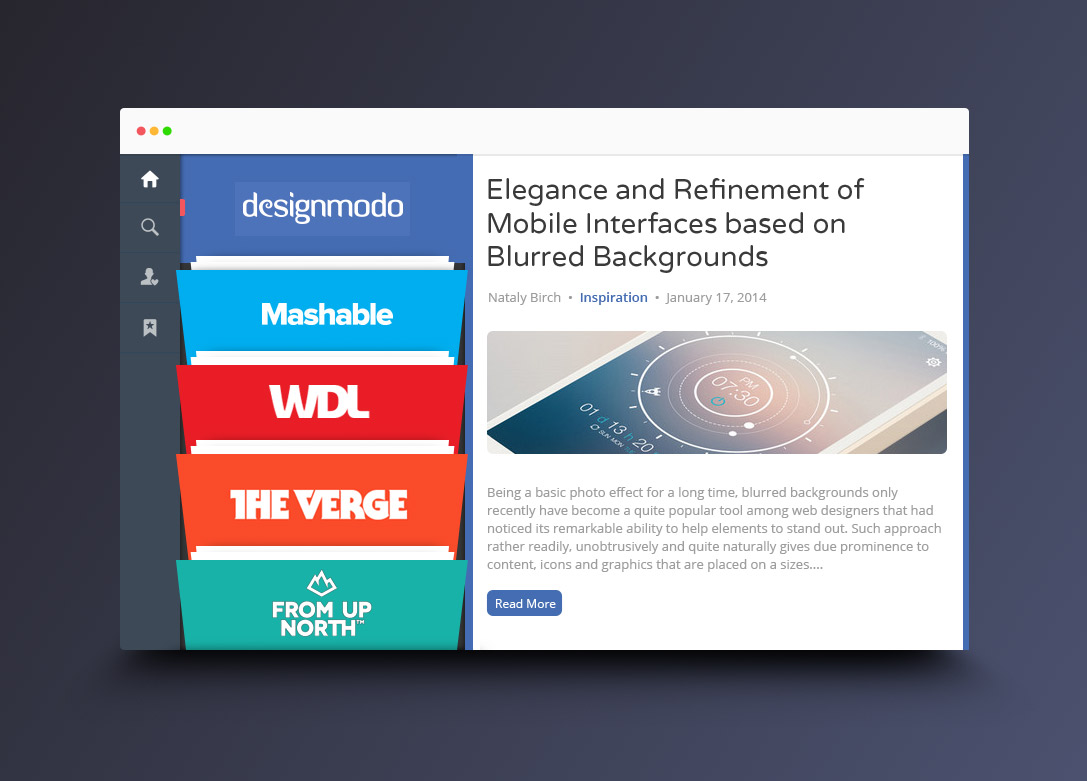The image depicts a screenshot of a website within a bordered frame. There is a dark blue boundary surrounding the main content, which showcases a website interface. On the left side of the website, there are five vertical listings of company names: Designmodo, Mashable, WDL, The Verge, and From Up North. On the right side of the website, there is an article titled "Elegance and Refinement of Mobile Interfaces Based on Blurred Backgrounds." In the upper left corner of the image, there are three colored dots — red, orange, and green — arranged horizontally from left to right. Additionally, there is a vertical banner featuring icons that represent a homepage, a search bar, a user profile, and a save icon.